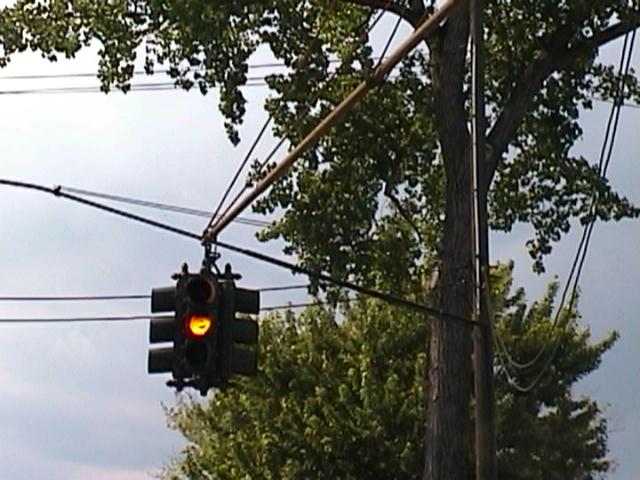The image captures a zoomed-in perspective of a black, old-fashioned intersection traffic light currently displaying yellow, indicating caution. The traffic light hangs freely from a thin pole, which is anchored in a manner typical of rural areas, making it susceptible to swaying in heavy winds. The light fixture itself has at least three visible sides, but the fourth side remains out of view. The scene includes the tops of two trees against an overcast sky, with one tree's prominent trunk positioned right behind the pole. No ground or street is visible in the tight frame, which focuses mainly on the traffic light and the sky beyond.